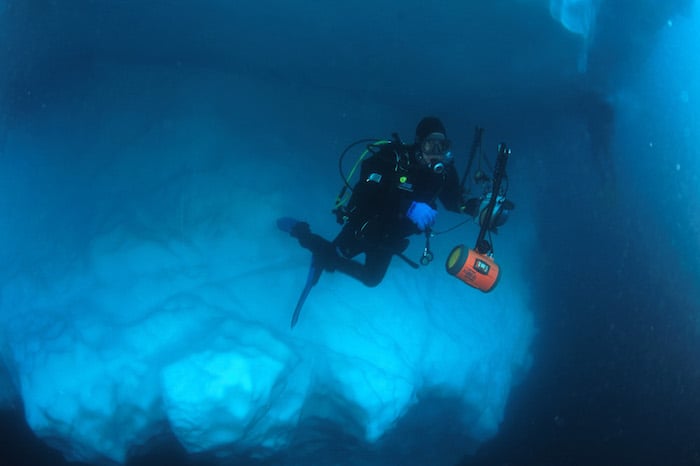This detailed, photographic-style image captures a scuba diver swimming toward the camera in an underwater setting. The diver's face is oriented toward the camera while his feet extend away. He is dressed in a black scuba outfit and wears blue gloves on his right hand. His left hand grips a pole with an attached orange cylinder that has indistinguishable text. The face mask resembles a yellow scuba tank. The scene behind him reveals a blue, luminous backdrop that includes what appear to be underwater caves, adding depth and intrigue to the setting. The upper and bottom right corners of the image transition into darker blue tones, contributing to the intense and somewhat eerie atmosphere. A potential additional diver is faintly visible in the background to the right, enhancing the scene's sense of depth and isolation. The image evokes a sense of profound solitude and adventure in the deep ocean.